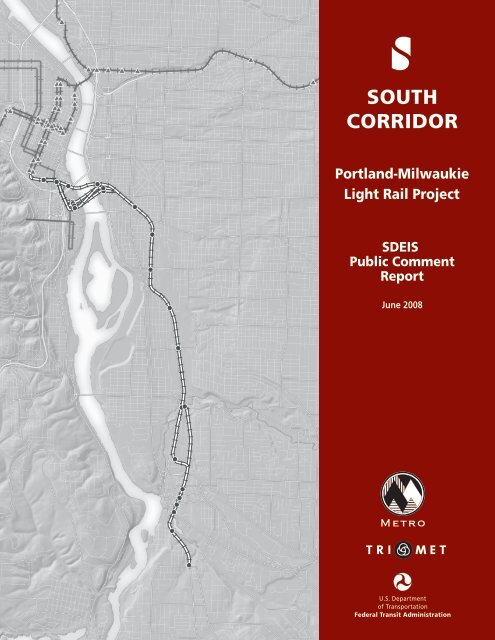The image displays the cover page of a public comment report titled "South Corridor, Portland-Milwaukee Light Rail Project, SDEIS, Public Comment Report, June 2008." The right side of the cover features a dark red bar with white text and logos. At the top is the title "South Corridor" accompanied by a distinctive double-sided "S" symbol. Below it, the report title and date are clearly listed. At the bottom of the red bar are three logos in succession: Metro, TriMet, and the U.S. Department of Transportation, Federal Transit Administration.

On the left side of the cover, there is an overhead map showing the design for the planned light rail project. The map is primarily gray, with the rail lines in black and white, crossing over a river that runs vertically through the map. The map itself is an outline of the city streets and does not contain additional labels or details.